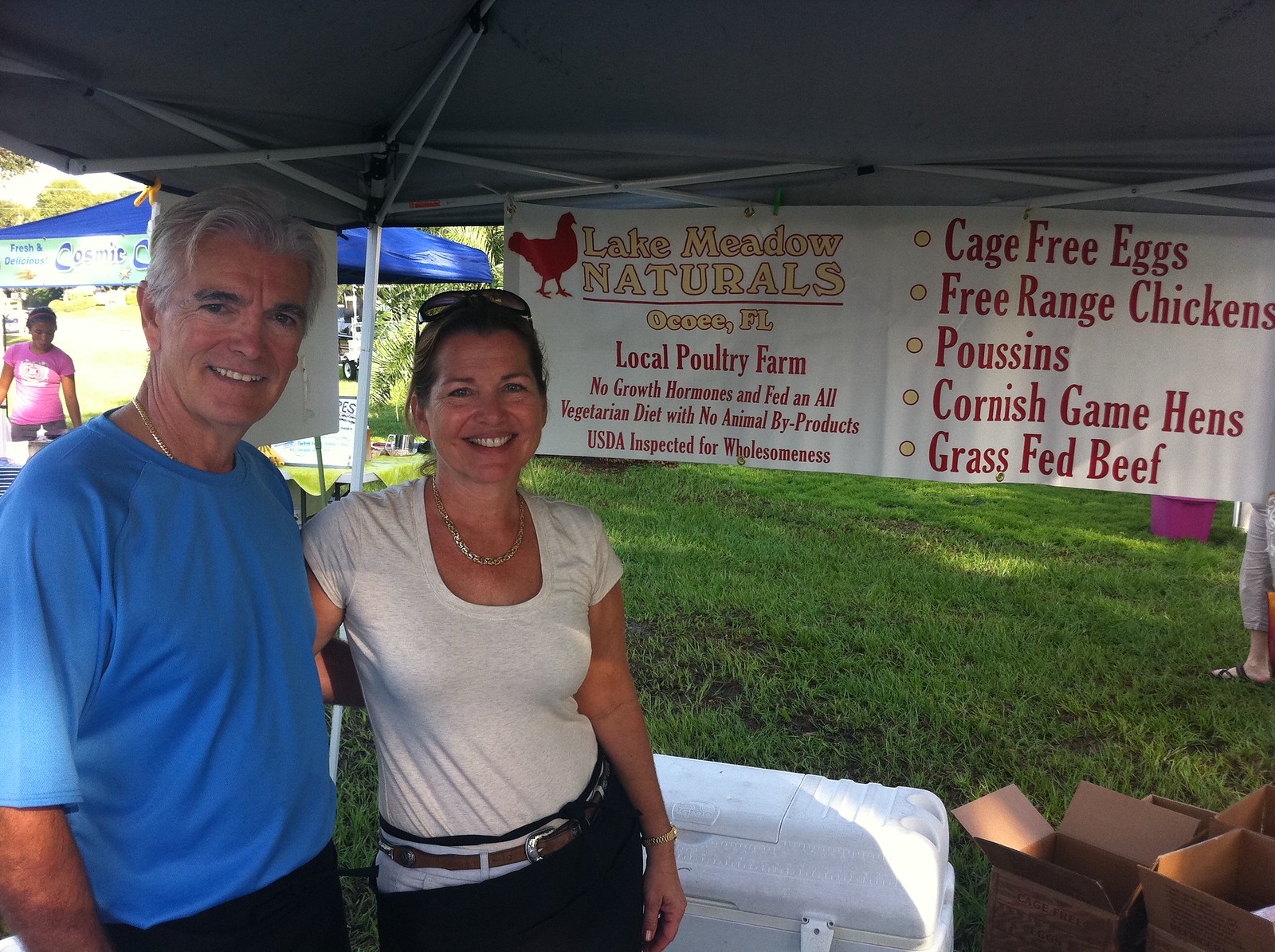In this vibrant image, we see a middle-aged couple at what appears to be a farmer's market or a food festival, standing under a white tent. The man, likely in his late 40s or early 50s with gray hair, wearing a blue polo shirt, gold necklace, and black pants, has his arm lovingly around the woman beside him. She is in her late 30s to early 40s, dressed in a white t-shirt, white jeans with a brown belt, possibly an apron, and sports brown hair with sunglasses perched on her head. They both might be wearing server's aprons, suggesting involvement in the event. 

Behind them is a prominent banner for Lake Meadow Naturals, featuring yellow text outlined in red that reads "Lake Meadow Naturals, Ocoee, Florida," alongside a red silhouette of a chicken. The sign emphasizes the local poultry farm's commitment to no growth hormones, an all-vegetarian diet, and USDA inspection for wholesomeness. Detailed bullet points advertise cage-free eggs, free-range chickens, poussin, Cornish game hens, and grass-fed beef. At their feet is a large white cooler and several open cardboard boxes, set on a grassy lawn. In the background, another tent is visible, along with a dark-skinned woman in a pink shirt looking down. This scene beautifully captures the bustling and communal atmosphere of the market.